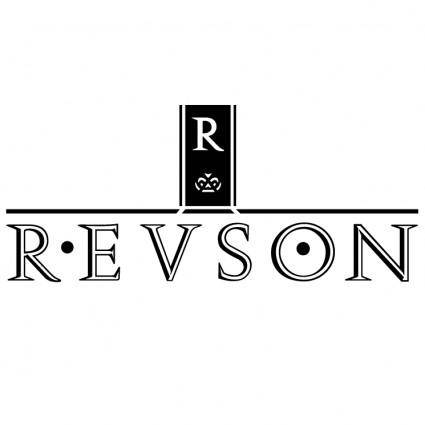This image features a minimalist, black-and-white logo set against a plain white background. Central to the design is a tall vertical black rectangle adorned with a large white capital 'R' at its summit. Directly below the 'R' is a white crown-like symbol, evoking a sense of elegance or royalty. The black rectangle itself is bordered on three sides—left, right, and bottom—by thin white stripes, but not on the top. Separating this central icon from the text below is a horizontal black line. Beneath this line, the word "Revson" is spelled out in prominent white letters, each outlined in black. Notable details include a black dot between the 'R' and the 'E', as well as another black dot in the center of the 'O'. The overall composition lends a sophisticated and regal air to the logo.